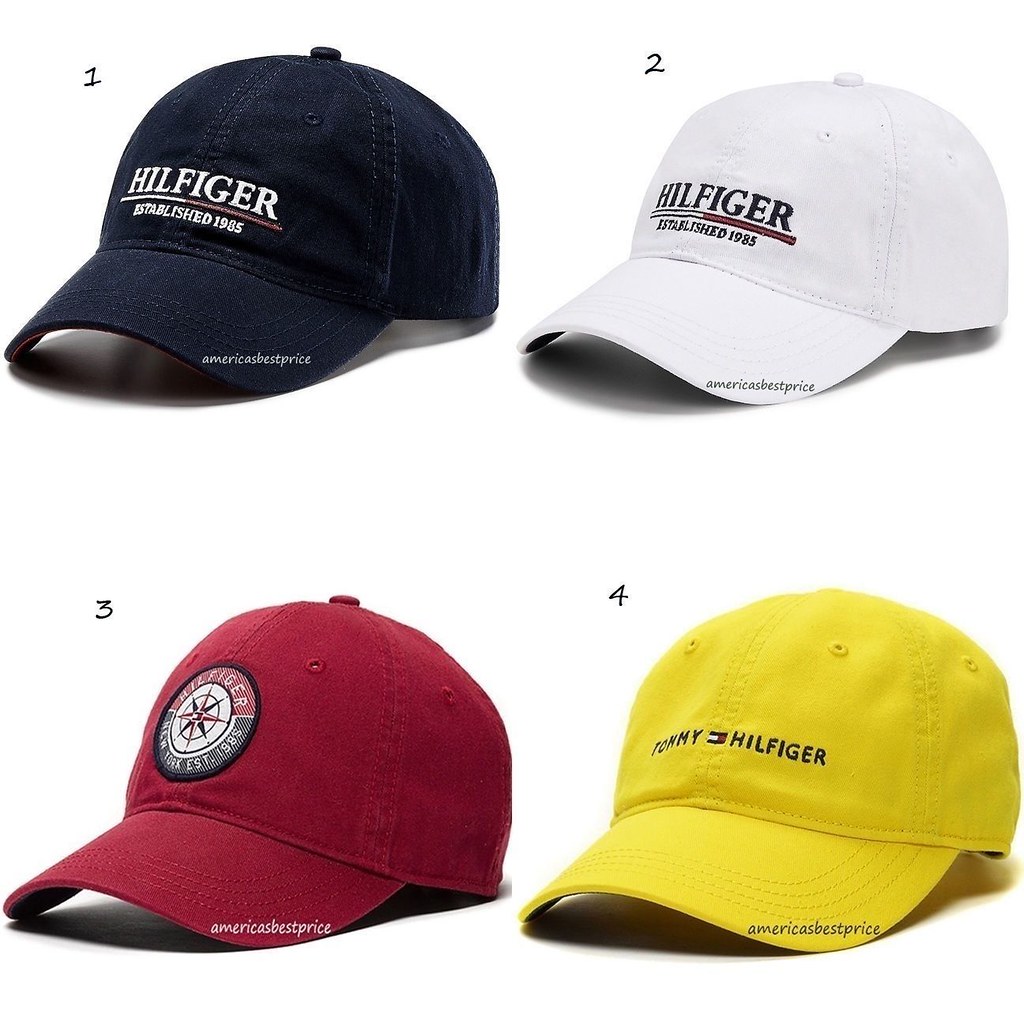In this photograph, we see four Tommy Hilfiger baseball caps, each numbered from one to four and set against a white background. All four caps are identical in shape, with curved bills, small circles for air ventilation, and a small button on top. The hats are labeled with numbers in black located at the lower left-hand corner of each.

- The first hat, numbered one, is dark blue with "Hilfiger" printed in white letters. It also features two intersecting lines, one white and one red, and is marked with "Established 1985" and "America's Best Price."

- The second hat is white and has "Hilfiger" printed in dark blue letters. It also reads "Established 1985," similar to the first hat.

- The third hat is red and features a circular patch with "Hilfiger, New York, Established 1985" and a star icon at the center. It also includes the phrase "America's Best Price."

- The fourth and final hat is bright yellow with "Tommy Hilfiger" written on it and includes a small red, white, and blue tag, sometimes referred to as the Hilfiger flag.

Each cap showcases distinct branding elements common to Tommy Hilfiger gear, providing a vibrant and varied selection of designs.